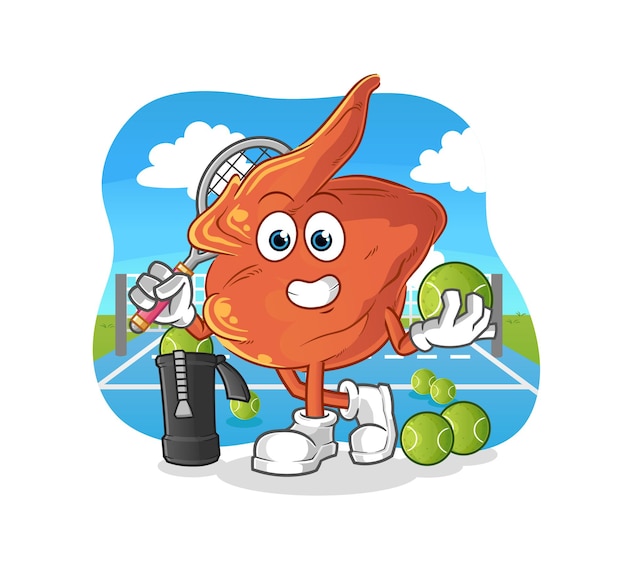The image features a whimsical cartoon character set against a backdrop of a blue sky filled with fluffy white clouds. The peculiar creature, resembling a blend between a pile of vegetables and a walnut, with suggestions of being a chicken wing, is primarily brown, orange, and yellow. It boasts a pointed peak that arches over its left eye. The character's face is animated with two large white eyeballs featuring blue and black centers, and a wide, white smile. It stands on spindly legs wearing cartoon-style white sneakers, reminiscent of Olive Oyl from the Popeye cartoons, accompanied by matching white gloves on its hands. The right hand, bent at the elbow, holds a tennis racket partially behind the body, while the left hand, with the palm facing up, grips a yellowish-green tennis ball. The character is positioned directly in the middle of a blue and white tennis court with additional tennis balls scattered around: one on the left and four on the right. Near its right arm, there's a black container with more tennis balls inside.